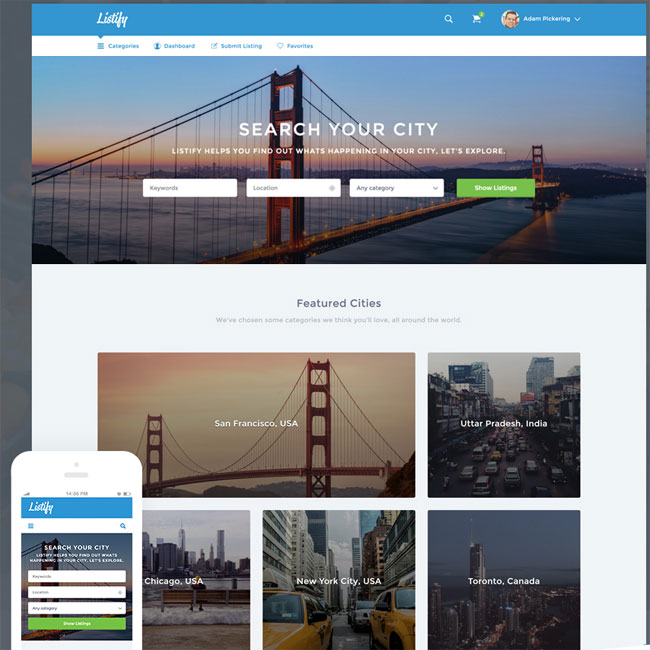This is a screenshot of a website that resembles Listly. The interface features a top navigation bar with various icons and options. Starting from left to right, it includes a search bar with a magnifying glass icon, a shopping cart icon, and a profile picture of a user named "Adam," followed by a drop-down arrow. Below this navigation bar is a thin white menu bar containing tabs labeled "Categories," "Dashboard," "Listing," and "Favorites."

Further down, there is an expansive banner featuring a search box overlaying a background image of what appears to be the Golden Gate Bridge in San Francisco. The text in white font within the banner suggests using the search feature to find out what's happening in your city, with a call-to-action that reads, "Let's explore."

At the bottom of this section, a label reads "Featured Cities," accompanied by five distinct image blocks, each representing different cities. The clean and structured layout aims to help users explore various locations and activities in their city seamlessly.